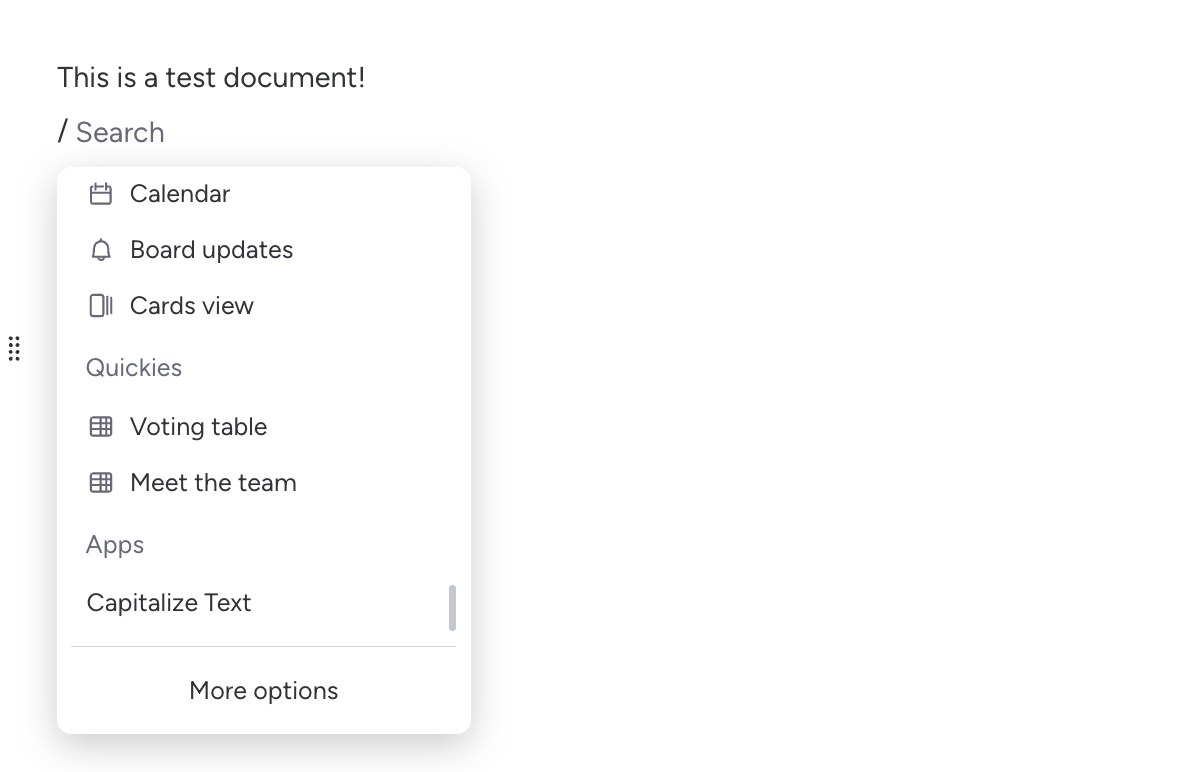The image displays a black-and-white screenshot of a pop-up box containing various options and information. At the top, it prominently states "This is a Test Document!" followed by "/search". Below this header, a list of options is provided:

1. "Calendar" accompanied by a calendar icon to the left.
2. "Board Updates" with a bell icon situated on the right.
3. "Card View" featuring a card icon on the left.

Further down, additional options are listed:
4. "Quickies"
5. "Voting Table" marked with a chart or grid icon to the left.
6. "Meet the Team" also represented with another grid icon to the left.
7. "Apps" followed by "CAPITALIZED TEXT" at the bottom.

At the very bottom of the list, the phrase "More Options on the Menu" is displayed.